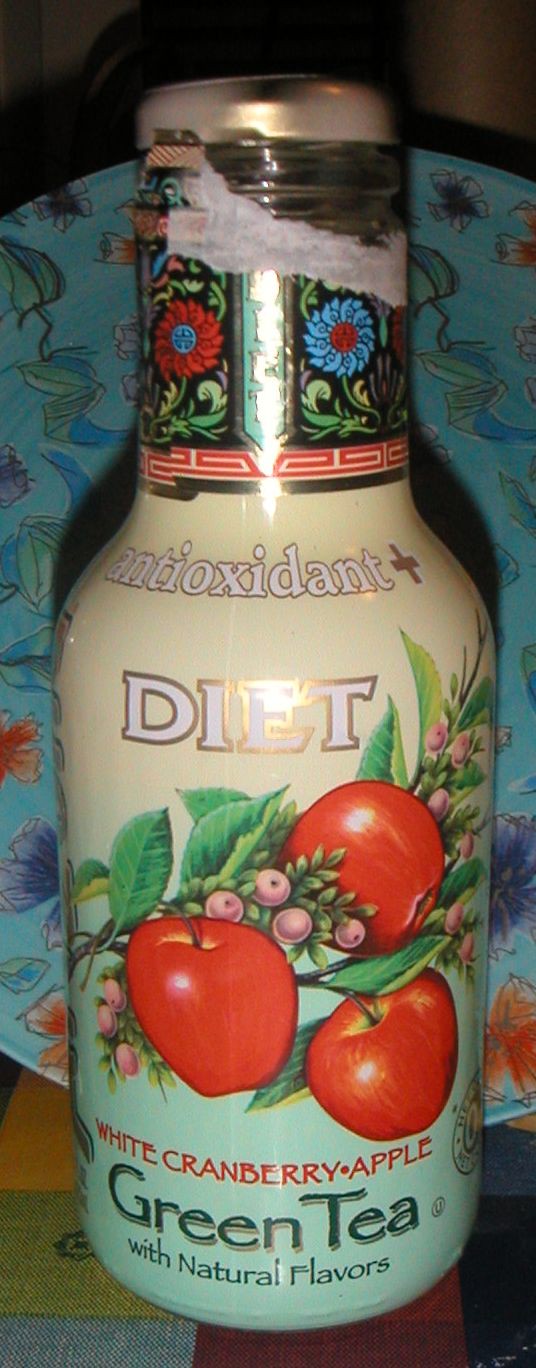In this color image, a prominently featured glass bottle sits on a plaid surface with its label facing outward. The bottle has a gold-colored cap with a white top, and just below the cap, the label shows a floral pattern with red and blue flowers. The label itself transitions from white to light green and displays detailed information: "Antioxidant Plus Diet" is written in bold text with gold trim, followed by "White Cranberry Apple" in red letters, and "Green Tea with natural flavors" in green text. The label also features a drawing of three red apples, light purple berries, and green leaves, though it is slightly torn at the top. In the background, there is a round, colorful dish with a light blue backdrop adorned with various leaves and flowers in purple, orange, and green.